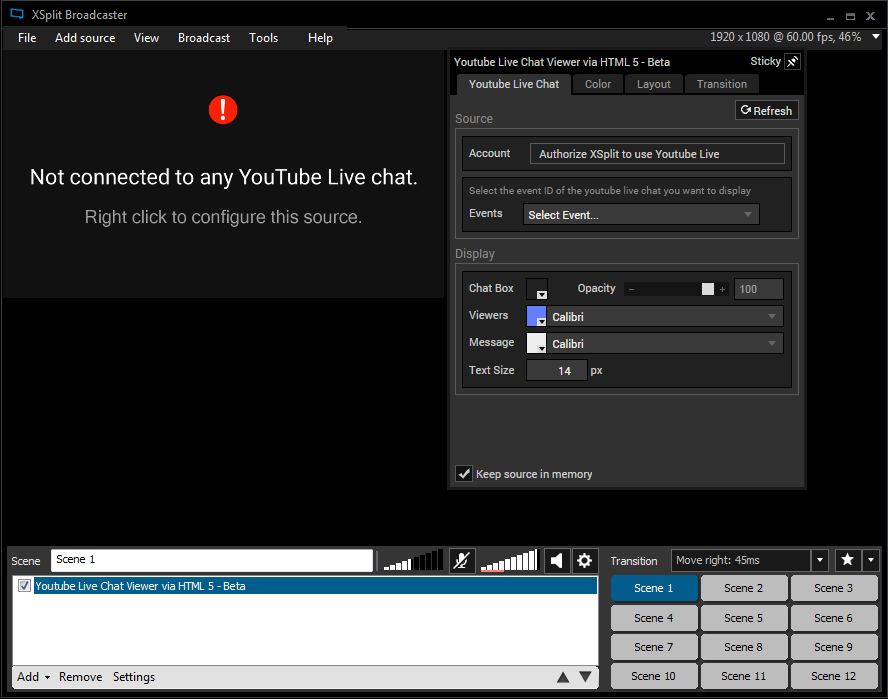The image is a screenshot from a desktop application, specifically XSplit Broadcaster. The interface is set against a black background. At the top of the window, there's a title bar labeled "XSplit Broadcaster". Below it, a menu bar lists various options: "File", "Add Source", "View", "Broadcast", "Tools", and "Help". Towards the far right of this bar, the display reads "1920 X 1080 at 60.00 FPS 46%", accompanied by a drop-down arrow.

Beneath the menu bar, on the left side, there is a notable alert symbol, a red circle with a white exclamation point, accompanied by the message "Not connected to any YouTube live chat. Right-click to configure this source."

On the right-hand side, a small pop-up window titled "YouTube Live Chat Viewer via HTML5 (Beta)" is open. This window features several tabs: "YouTube Live Chat", "Color", "Layout", and "Transition", with the "YouTube Live Chat" tab currently selected. The content under this tab reads:

- Source
- Account
- Authorize XSplit to use YouTube Live
- Select the event ID of the YouTube Live Chat you want to display.

Below these instructions is a drop-down menu labeled "Select Event". Further down, another section named "Display" contains options for "Chat Box", "Opacity", "Viewers", "Message", and "Text Size". This screenshot offers a comprehensive look at the interface settings and configuration options for integrating YouTube Live Chat within XSplit Broadcaster.